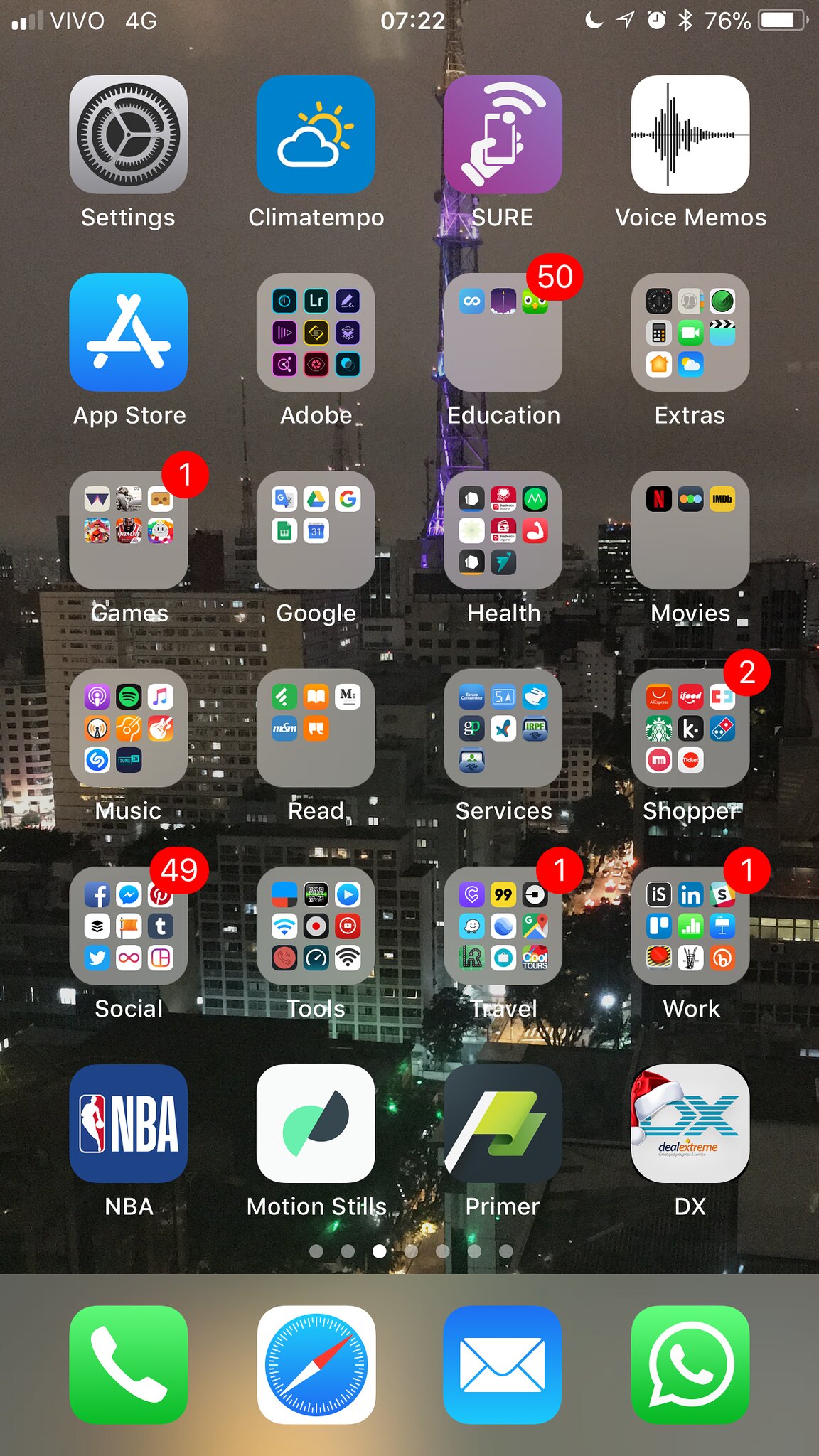The iPhone screenshot showcases a densely packed home screen, with a plethora of app icons spanning the entire display. The wallpaper is completely obscured by these icons, indicating that the device owner has a vast collection of apps. The apps are partially organized into groups: one for Adobe, another labelled Extras, Read, Music, Services, and more, with each group containing multiple applications. Among the ungrouped icons are essential utilities like Settings, Climate, Tempo, Voice Memos, App Store, NBA, Motion Stills, and Primer DX.

At the bottom, the dock contains the most frequently used apps including Phone, Safari, Mail, and FaceTime or possibly Messages. The Social folder, filled with popular platforms such as Facebook, Twitter, Pinterest, and Tumblr, prominently displays 49 unread notifications. Another folder named Education, which includes apps like Duolingo, shows 50 unread notifications. This chaotic yet somehow structured array of applications emphasizes the extensive digital toolkit maintained by this user.